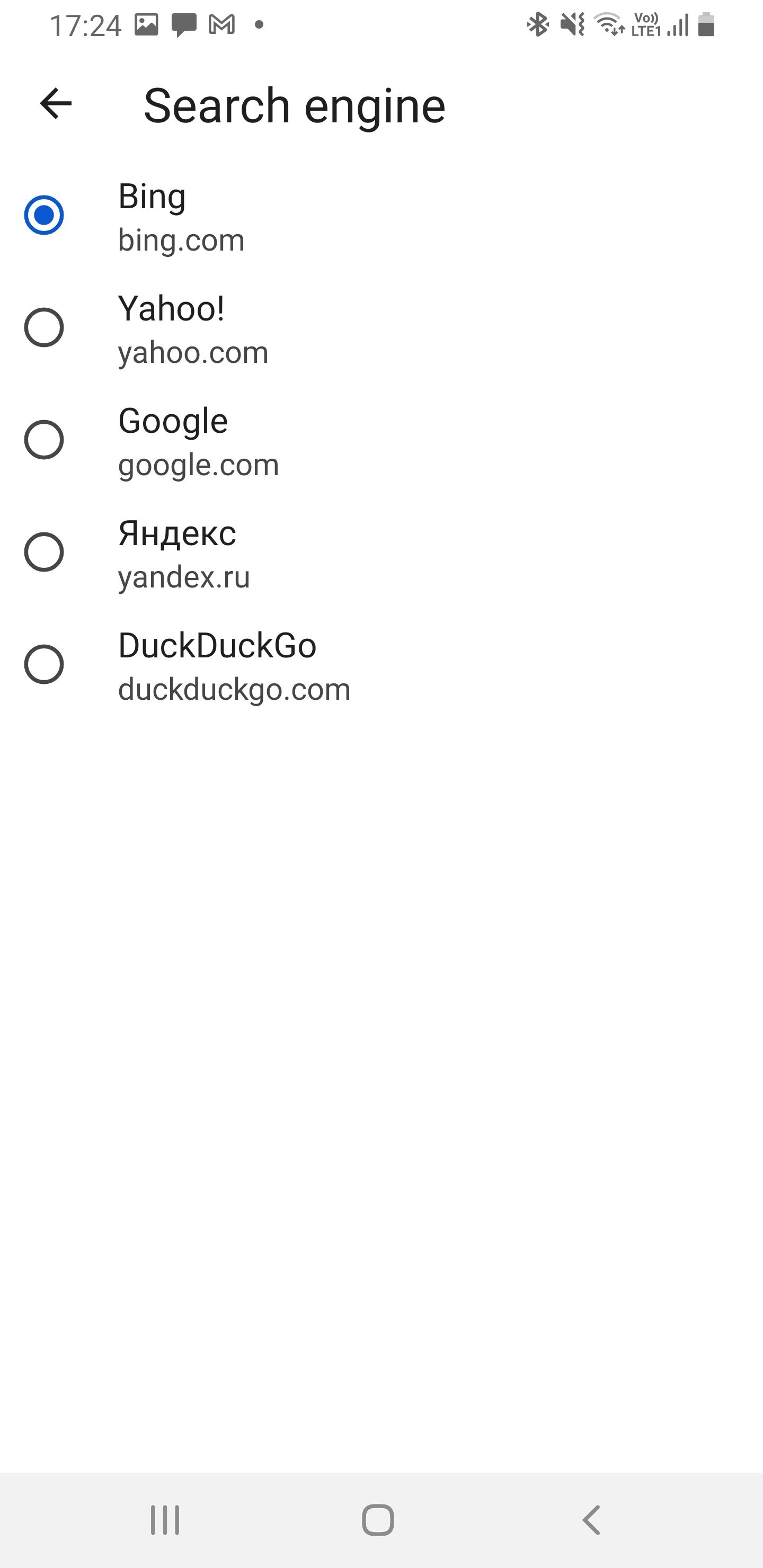A vertically-oriented screenshot from a smartphone displays a settings page, where the user can select their default search engine. At the top of the screen, the status bar includes various icons: a picture icon, a speech bubble, a mail icon represented by the letter 'M', and a black dot. The right-hand side of this bar shows connectivity and status indicators, including Bluetooth, silence mode, Wi-Fi signal, and battery level.

The main content of the page is set against a white background. At the top left, a back arrow is visible beside the bold title "Search Engine." Below the title, five selectable options are listed in smaller font, each accompanied by a circular radio button. The choices include Bing, Yahoo, Google, a search engine in Cyrillic script, and DuckDuckGo. The option for Bing is highlighted with a blue-filled circle, indicating it is the currently selected search engine, while the others remain unselected.

At the bottom of the screen, the Android navigation menu features three icons: a set of horizontal lines for navigating tabs on the left, a circular home button in the center, and a back arrow on the right.